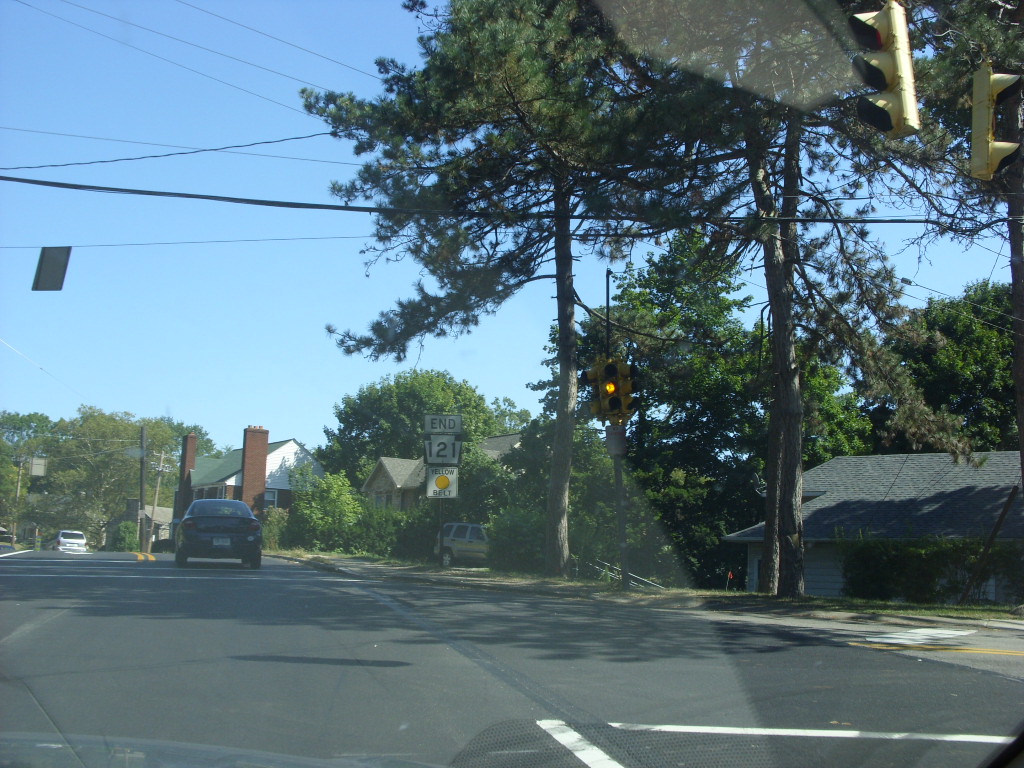In this image, we are looking out of a car window onto a quiet neighborhood street. The scene is detailed with two traffic lights situated in the right-hand corner of the photo and a corner light mounted on a pole almost at the center. Positioned near the middle, there's a prominent street sign indicating "End 121." The right side of the road is shaded and lined with homes nestled among a dense array of trees. One of the homes in the distance features a distinct brick chimney. Further back in the background, a white car can be seen on the far left-hand side of the image. In the middle ground, under the shade of a tree, an indiscernible colored sedan is parked. Lastly, a light brown minivan is visible in a driveway, nestled among the houses' greenery.